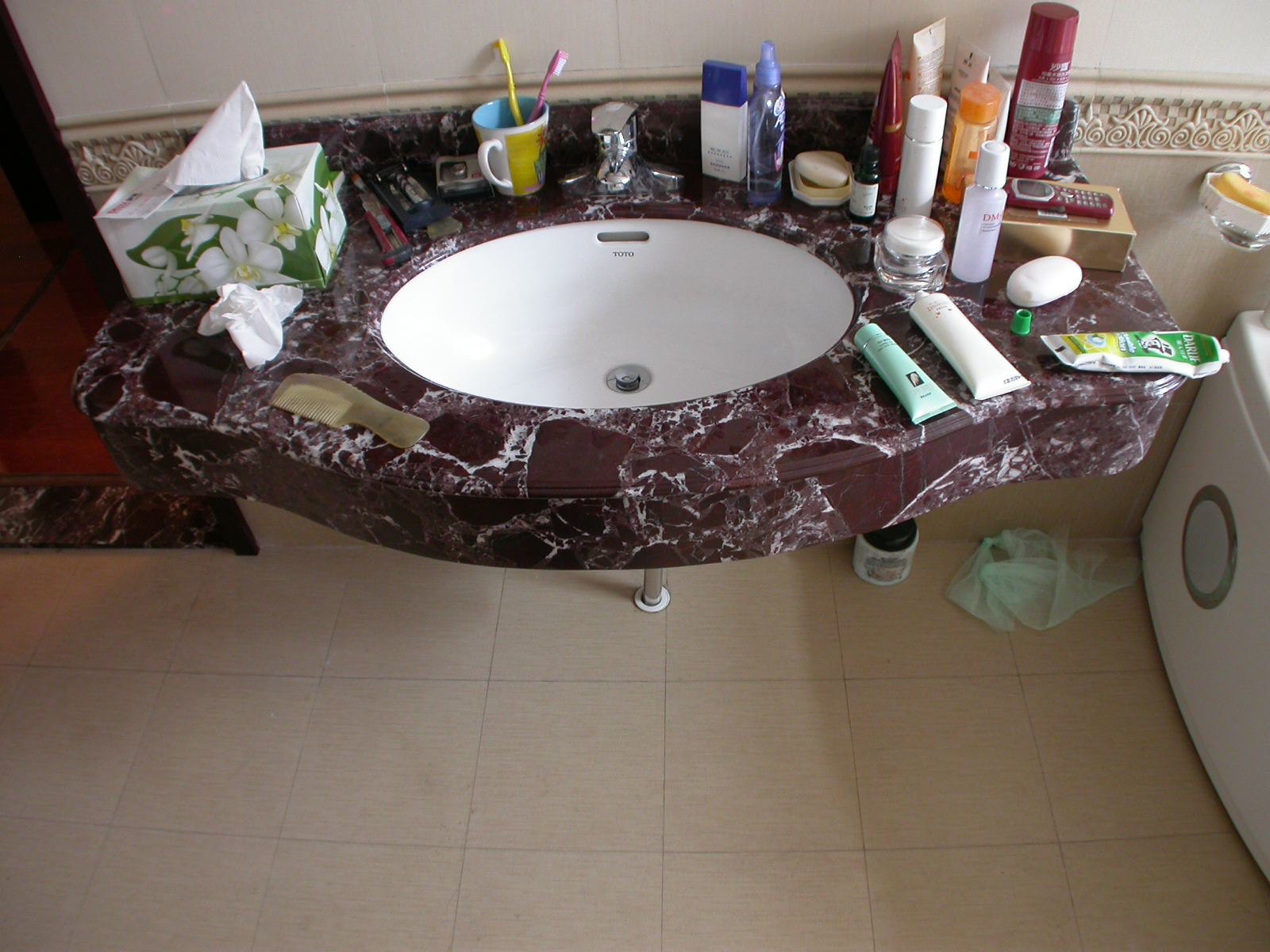The photo showcases a detailed bathroom vanity setting. The floor is adorned with whitish-tannish tiles, providing a clean and neutral backdrop. The vanity top stands out with its striking dark brownish-reddish hue and elegant white marbling. Prominently displayed is a decorative tissue box featuring green leaves and white flowers. 

On the counter, there are two packs of toothpaste and two toothbrushes still in their packaging. A used tissue lies in front of the tissue box, and nearby is a brown comb with a handle. A coffee mug holds two toothbrushes, one yellow and one pink. 

Additionally, there is a bottle of cologne and another clear bottle—contents unclear but possibly hand soap. An old-fashioned cell phone, reminiscent of models from 2005 or 2006, rests on a wooden box. Scattered around are a tube of toothpaste, a clear short jar, a container of essential oils, and what seems to be a can of shaving cream.

In the background, the edge of a bathtub is just visible, hinting at the rest of the bathroom space not fully captured in the frame.